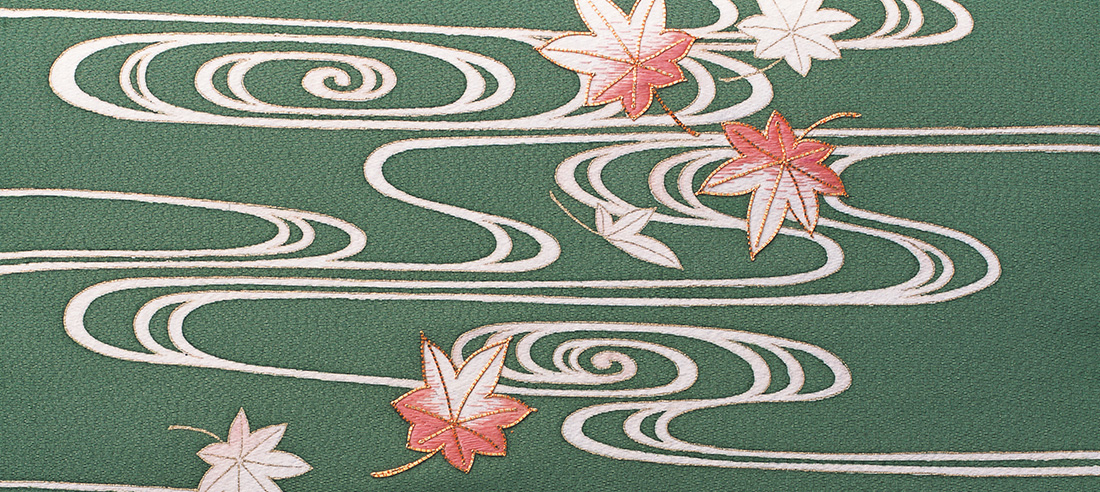This rectangular landscape image, approximately five inches wide and two inches high, showcases what appears to be a section of fabric or wallpaper with a predominantly light forest green background. The backdrop features intricate, river-like white lines that swirl and spiral across the entire surface, starting from the upper left corner and branching off in various directions. Interspersed among these flowing patterns are several leaves, specifically five in total. Three of these leaves display a unique color gradient, with the lower part in a pinkish-orange shade transitioning to white, and they appear to have delicate gold stems. The remaining two leaves are entirely white. The leaves, resembling seven-pointed maple leaves, seem to be artistically scattered, giving the impression of them gently falling across the material. Together, these elements create a textured and visually engaging design.